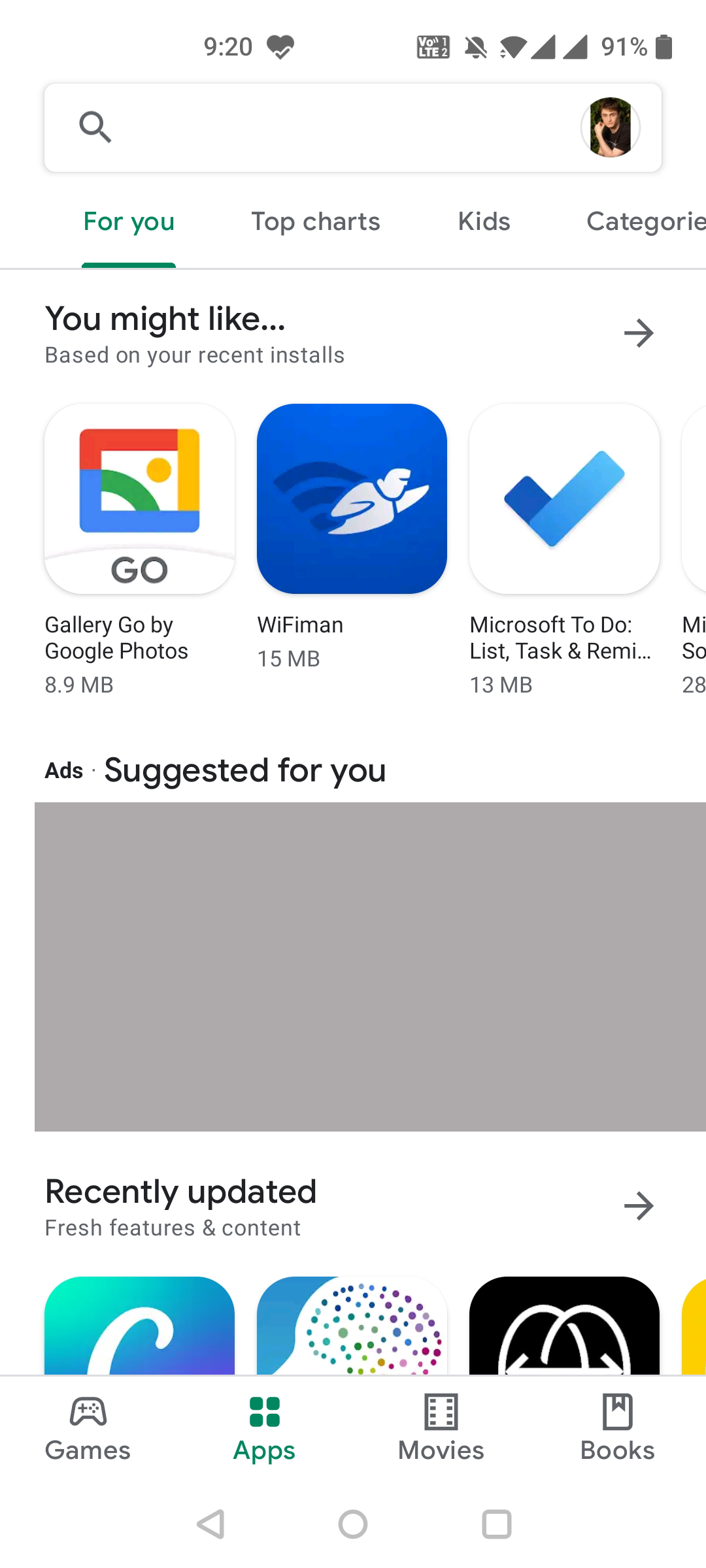This image is a screenshot from a smartphone displaying the Google Play Store interface, set against a white background. At the top of the screen, the time is shown as 9:20, and the battery icon on the right side indicates a 91% charge. Below this, there is a prominent search bar featuring a search icon on the left and a partial profile photo of an individual. The profile picture reveals the person's left arm and part of the face, but it is too obscured to determine distinct features, though the individual appears to be either Caucasian or Asian.

Directly beneath the search bar, the navigation tabs display various categories. The tab "For You" is highlighted in blue, while "Top charts," "Kids," and "Categories" (with the "S" partially cut off) are shown in gray. Under this navigation menu, there is a bold, gray header stating "You might like" followed by the text "Based on your recent installs."

The suggested apps listed include:
1. "Gallery Go by Google Photos" 
2. "Wi-Fi Man," whose icon is a blue square with rounded corners featuring a cartoon character.
3. "Microsoft To Do," with an icon depicting a white box and a two-tone blue checkmark.

There is also a section labeled "Ads" with the text "Suggested for you," but the actual advertisement content is obscured, appearing as a light gray rectangle. At the bottom of the screen, the partially visible "Recently updated" section shows the upper halves of app icons.